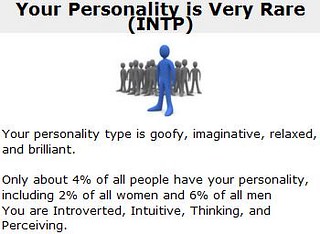The image is a square, digital illustration with a white background, designed to resemble a slide. At the top, a light gray banner features bold, black text stating, "Your personality is very rare," with "INTP" enclosed in brackets beneath it. Centrally, the illustration contains a simple, blue outline of a person standing prominently in front of a group of gray-outlined individuals, symbolizing uniqueness and distinction. Below the image, black text describes the personality type as "goofy, imaginative, relaxed, and brilliant." A paragraph at the bottom adds further detail, noting that only about 4% of all people have this personality type, with a gender breakdown of 2% of all women and 6% of all men. The text also identifies these individuals as being introverted, intuitive, thinking, and perceiving. The entire composition is neatly laid out against a clean, white background, giving the image a clear and polished appearance.